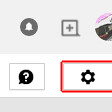The image being described is a very small, cropped square from a computer screen capture, primarily showcasing a portion of a menu bar. At the top of this square, a slightly gray background is visible. Positioned on this background, towards the left, is a small, dark gray circle featuring a white bell icon.

Just off-center to the right of this bell icon, there is a dark gray square shape with a small line extending from its bottom right corner and a plus sign in its middle. Further to the right, partially cut off by the image boundary, is another circle displaying what appears to be a user's icon, adorned with pink, brown, and white colors.

The middle section of the image contains a white rectangular space, within which several interactive elements are displayed. On the left side of this space is a square-shaped box containing a black speech bubble with a white question mark inside it. To the right of this speech bubble icon is a red-outlined rectangle with a black gear symbol centered within it.

At the bottom of the image, there is another strip of dark gray space, completing the cropped visual representation of the computer menu bar.